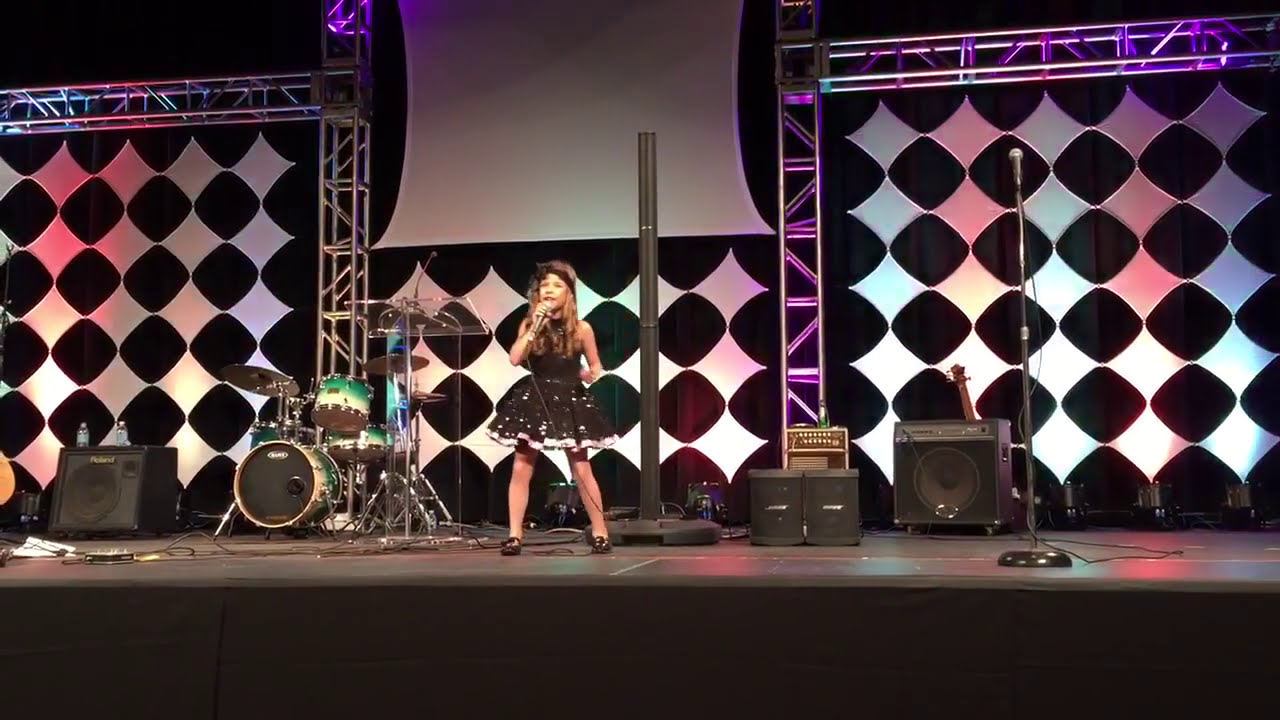In the image, a young girl, approximately 11 or 12 years old, stands at the center of a stage, holding a microphone and appears to be singing. She is dressed in a cute black dress with floral designs and a white accent stripe at the bottom, which falls just above her knees. Her long, curled, blondish-brown hair cascades down past her chest, complemented by a black headband. She wears tan stockings and shiny black shoes.

The stage around her is cluttered with various musical equipment. Directly behind and to her right is a drum kit with green-tinted sides, and further to her right stands a large speaker and a resting bass guitar. To her left, there are several smaller speakers, another large speaker, and an additional microphone stand. Wires are scattered around the stage floor, hinting at the equipment setup necessary for a concert venue.

The backdrop features a black and white diamond pattern interspersed with rounded black squares, adding a dynamic element to the scene. There are also metal accessories that stretch from the floor toward the ceiling, flanking from the center and extending to both sides of the stage, enhancing the structural aesthetics. There is no visible text in the image, but the array of colors including black, brown, silver, green, purple, pink, and white adds to the vibrant atmosphere of the performance setting.